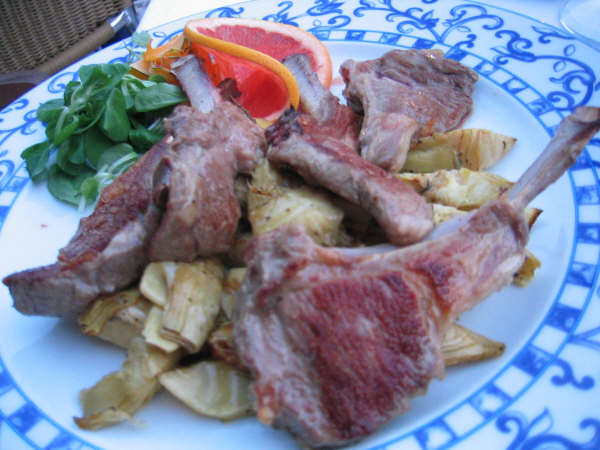This photograph captures a close-up, slightly angled left-side view of a plate of food taken outdoors, perhaps during sunset or on a cloudy day. The plate, which is round with a white center and a blue and white border featuring a subtle swirl and striped pattern with floral accents, prominently displays four browned pork chops. The pork chops, with their bones pointing out, are neatly arranged atop a substantial bed of thick-cut French fries or possibly potatoes and onions. Toward the back left of the plate, there’s a vibrant twisted slice of grapefruit, orange on the outside and bright red inside, beside a small pile of fresh green leaves, likely watercress or spinach, that appear moist. In the background, a wicker chair is partially visible in the upper left corner, contributing to the outdoor dining ambiance.